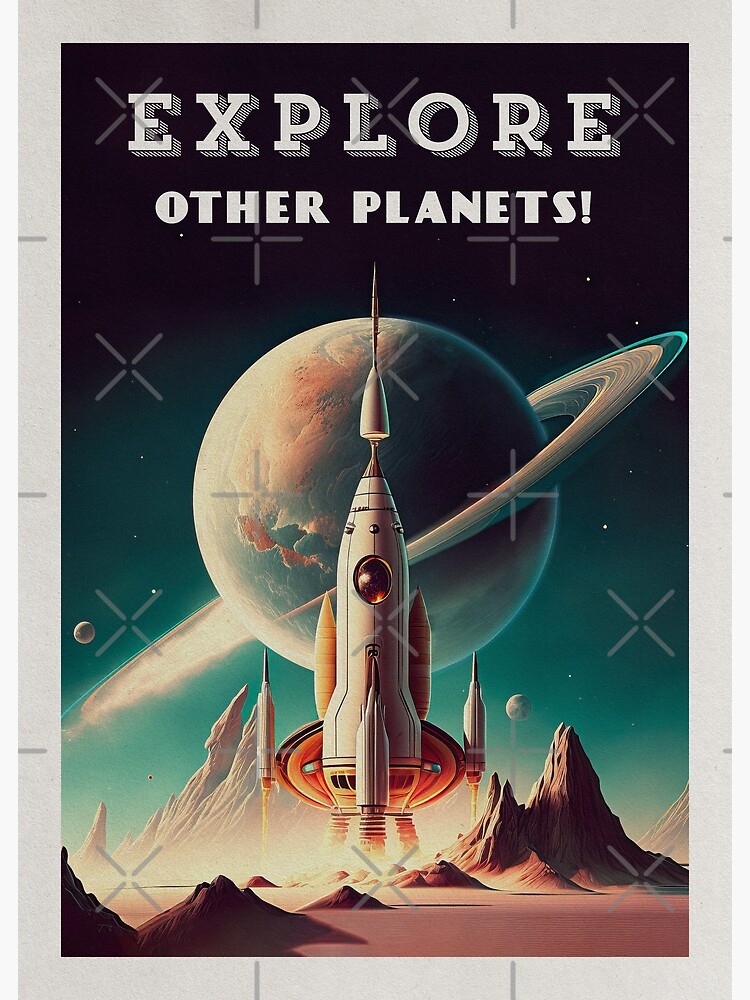The image is a vibrant digital art piece styled like a vintage travel poster with a science fiction twist, reminiscent of the 1950s Jetsons era. At the top, the bold white text "EXPLORE" is prominently displayed, followed by "OTHER PLANETS!" in eye-catching letters. The background presents a mesmerizing ombre gradient transitioning from deep black to various shades of blue, adorned with stars, creating a captivating space theme. Central to the image is a striking depiction of Saturn, easily recognizable by its iconic rings, though the colors present a unique blend of very light blue and orange. In front of Saturn, a futuristic rocket ship with a tall pointed spire is either taking off or landing, featuring a circular window and multiple miniature thrusters. Below the rocket, the ground showcases rugged, sandy-colored mountains, implying an alien landscape. In the background, other planets are faintly visible, enhancing the space exploration theme. Overlaid across the entire image are subtle, translucent X's and plus signs, adding a technical, science fiction nuance.